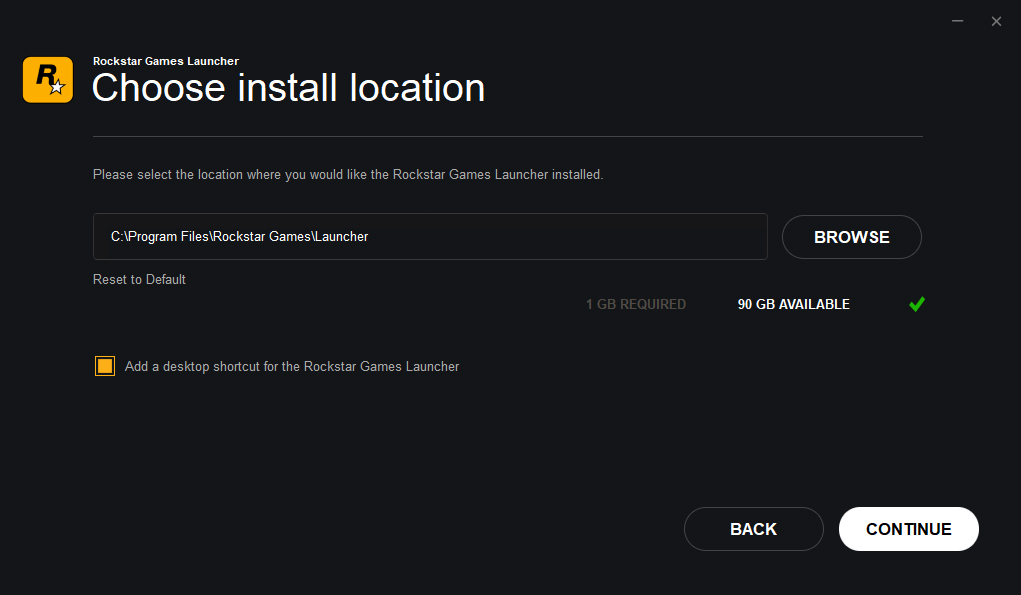The image displays a dark mode screen, primarily using a deep black or possibly navy blue background. Central to the image is information pertaining to the installation of a game launcher. In the upper left corner, an orange icon featuring an "R" with a star at the base of the letter is prominently displayed, indicating the Rockstar Games logo. Next to the logo, white bold text reads "Rockstar Games Launcher."

Below this title, a directive in gray asks users to "Please select the location where you would like the Rockstar Games Launcher installed." Just beneath this instruction is a text input field prefilled with "C:\Program Files\Rockstar Games\Launcher," indicating the default installation path. To the right of the text field is a "Browse" button for users to choose an alternative location.

Further down, the screen notes "Reset to default," followed by specifications of "1 GB required, 90 GB available," accompanied by a green checkmark ensuring enough storage is available. An orange checked box below this section reads, "Add a desktop shortcut for the Rockstar Games Launcher."

At the bottom, navigation options include a black "Back" button on the left and a white "Continue" button on the right.